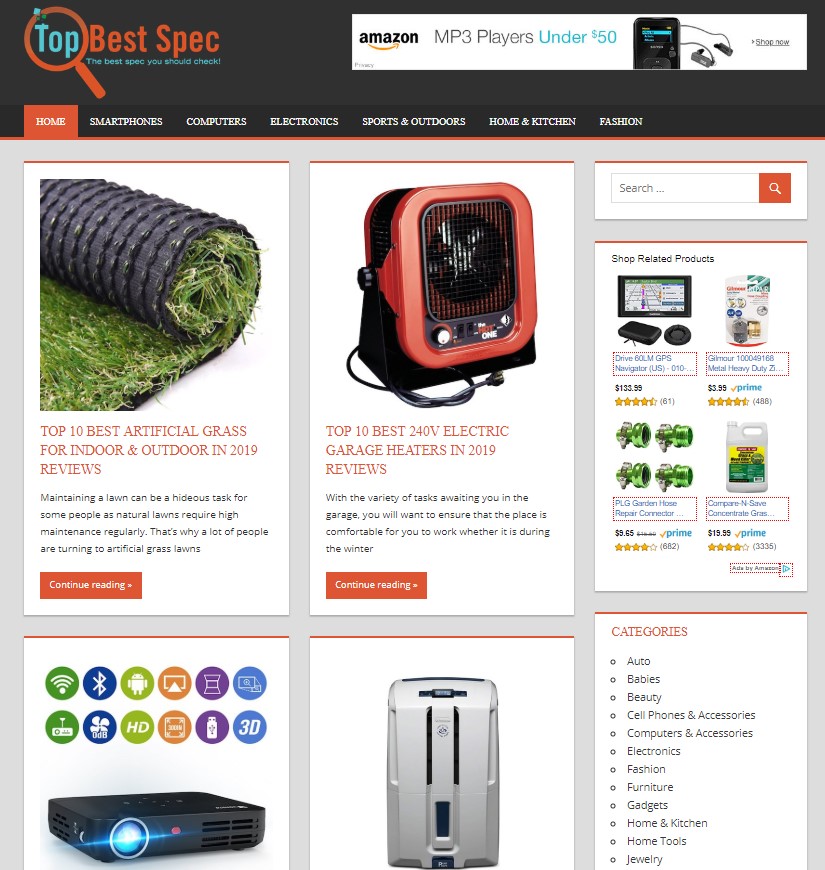In the vertically-oriented rectangular image frame, we are presented with a screenshot of a website titled "Top Best Spec." The site boasts the tagline "The Best Spec You Should Check" prominently in the top left corner. To the right of this, an Amazon MP3 player advertisement is visible. 

Directly below these elements, a navigation bar displays active and inactive selection options including: "Home" (currently active), "Smartphones," "Computers," "Electronics," "Sports & Outdoors," "Home & Kitchen," and "Fashion."

Beneath the navigation bar, the screen is divided into three columns. The left and middle columns are slightly wider and feature individual product listings. In the left column, there is a listing titled "Top Ten Best Artificial Grass for Indoor and Outdoor in 2019 Reviews." The middle column features a listing for the "Top Ten Best 200 Volt Electric Garage Heaters in 2019 Reviews." Both listings are accompanied by images of the respective products.

The narrower right column includes a continuation of product listings, though not fully visible in the frame. The bottom of the image displays two more products, partially cut off, with images only. One appears to be a projector, and the identity of the other product remains unclear.